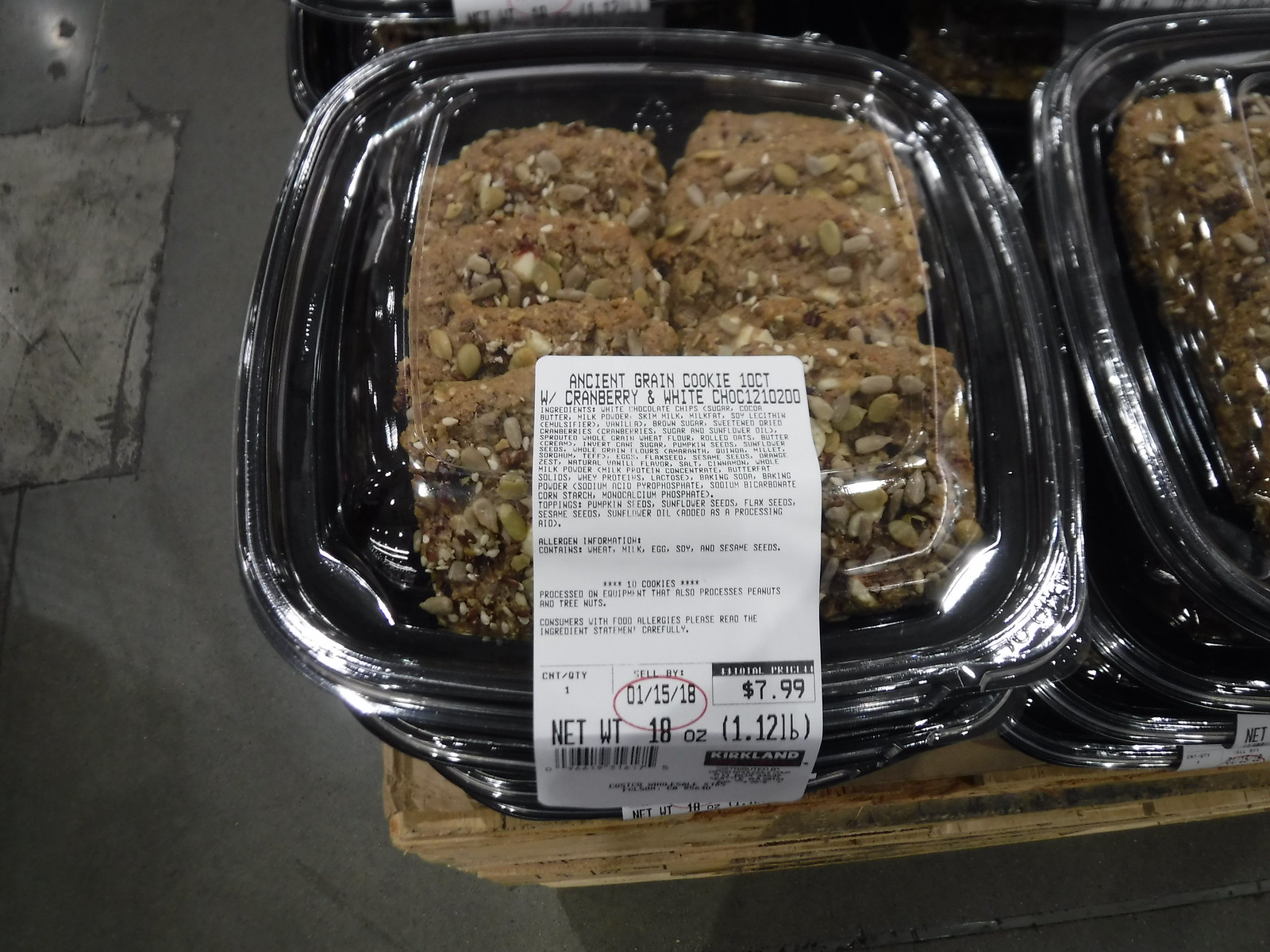The image captures a detailed, close-up view of two stacks of cookie tubs placed on a brown wooden table. Each stack comprises three transparent tubs containing healthy ancient grain cookies in a cranberry and white chocolate flavor. The tubs are made from black plastic with clear plastic lids, secured with receipt tape over the side. The price of the cookies is clearly visible at $7.99. In addition to the pricing, there is a long list of ingredients prominently displayed on the tubs. The setting is illuminated by bright lighting that reflects off the clear plastic lids, adding a touch of shine to the scene. The background features a gray slate floor, viewed from an overhead perspective.